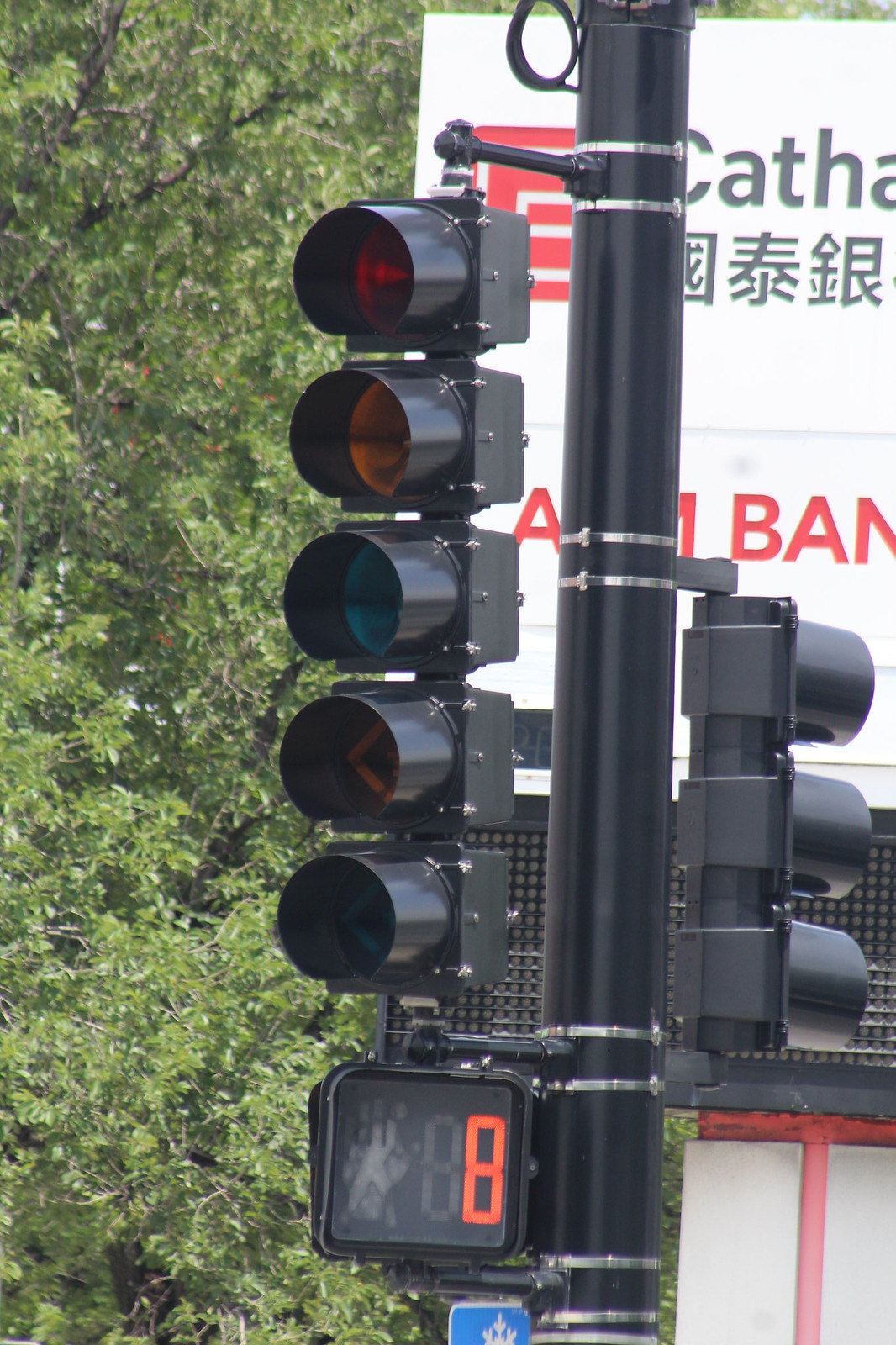The image depicts an outdoor scene centered around a traffic light setup at a pedestrian crossing. Dominating the foreground is a black light post, featuring an electronic timer displaying an orange "8," indicating the seconds left for pedestrians to safely cross the street. The traffic light configuration on the pole is unconventional, with four lights on one side and three on the other. In the background, to the left of the frame, lush green trees with visible branches fill the area, providing a natural contrast to the urban environment. On the right, a white billboard marked with partial English letters "C-A-T-H-A" and Chinese characters is prominently displayed. Below the Chinese text, red letters spell out "A-B-A-N." The scene captures the intersection of nature and city life, highlighting the functionality of the traffic system and the surrounding visual details.